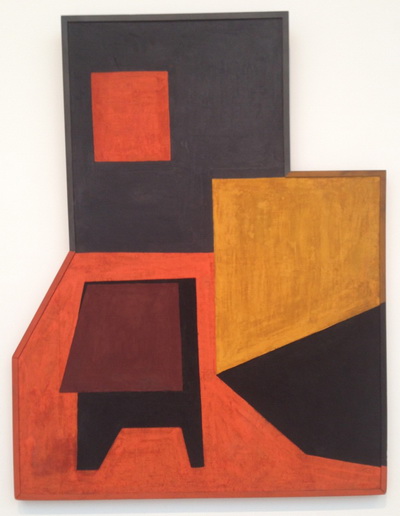The painting is a geometric composition set against a very light pink background, which evokes the style of Cubism. At the top center of the image, there is a large gray square, within which there is a smaller orange square occupying about half the dimensions of the larger gray square. This arrangement resembles a stylized door with a doorknob. Below this central gray square, an orange block extends downward, covering a portion of the lower area—possibly signifying a floor. On this orange area, there is a brown table or desk with black legs. To the right, a slanted lighter brown shape, possibly resembling a counter or front desk, casts a black shadow beneath it. Additionally, there is a yellow square with an outward extension and some black markings beneath, which could be interpreted as table legs. This intricate arrangement of shapes and colors collectively evokes an abstract depiction of a room or office.